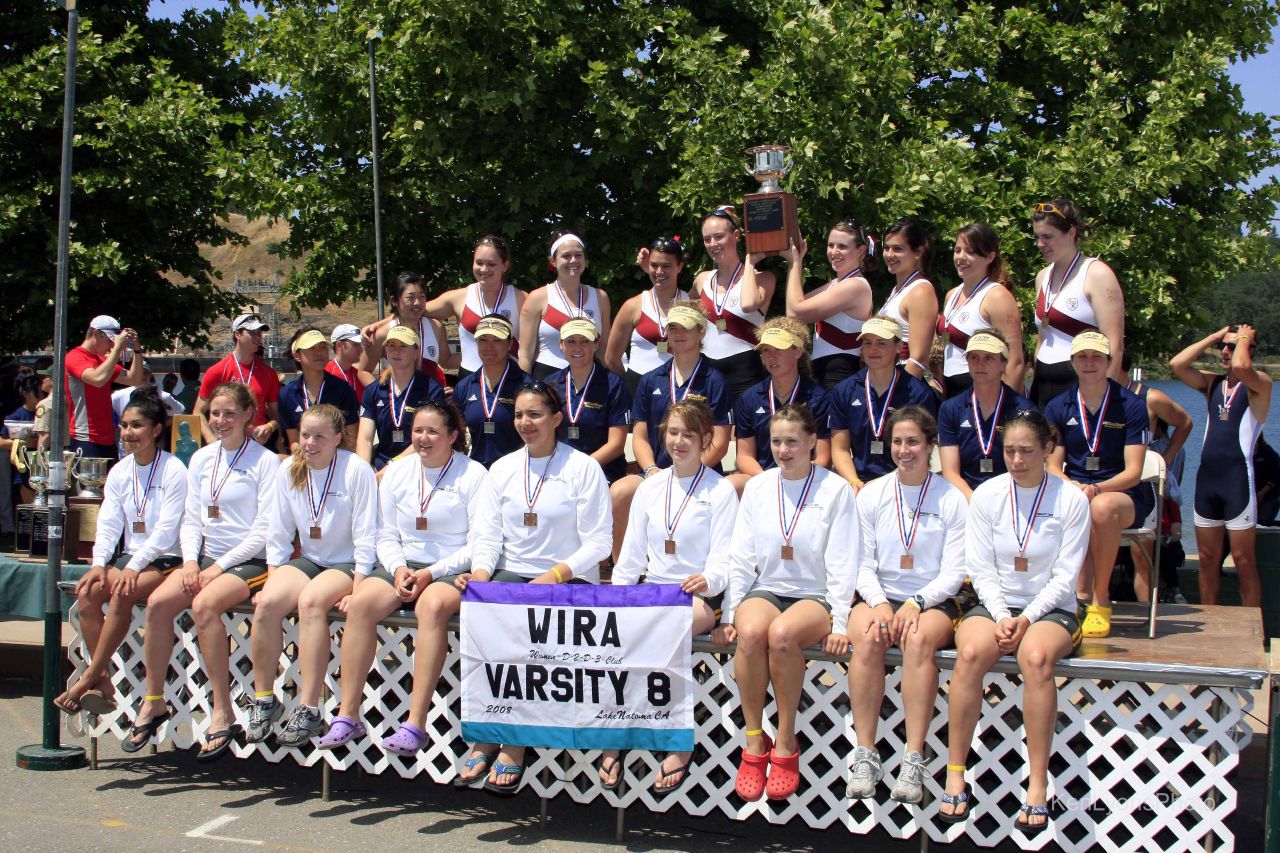In this vibrant outdoor scene, a group of varsity club young women are arrayed on a three-tiered platform. At the forefront, several women clad in white long-sleeved tops and shorts dangle their bare legs over the edge of the stage, displaying medals around their necks. They hold a sign reading "WIRA Varsity 8" with purple and black lettering. Behind them, a second row of women in blue shirts and shorts are seated on chairs, also sporting medals. The backdrop features a final row of women standing, wearing a mix of white, red, and blue tops, along with striking white glasses with a dark red horizontal stripe. Among this standing group, two central figures proudly hoist a large trophy with a wooden base and a gleaming silver cup. Flanking the group to the left, two men in red shirts add a contrasting visual element. The entire ensemble is set against a scenic outdoor backdrop, complete with lush trees, a serene body of water to the right, and rolling hills to the left, capturing a moment of athletic triumph and camaraderie.